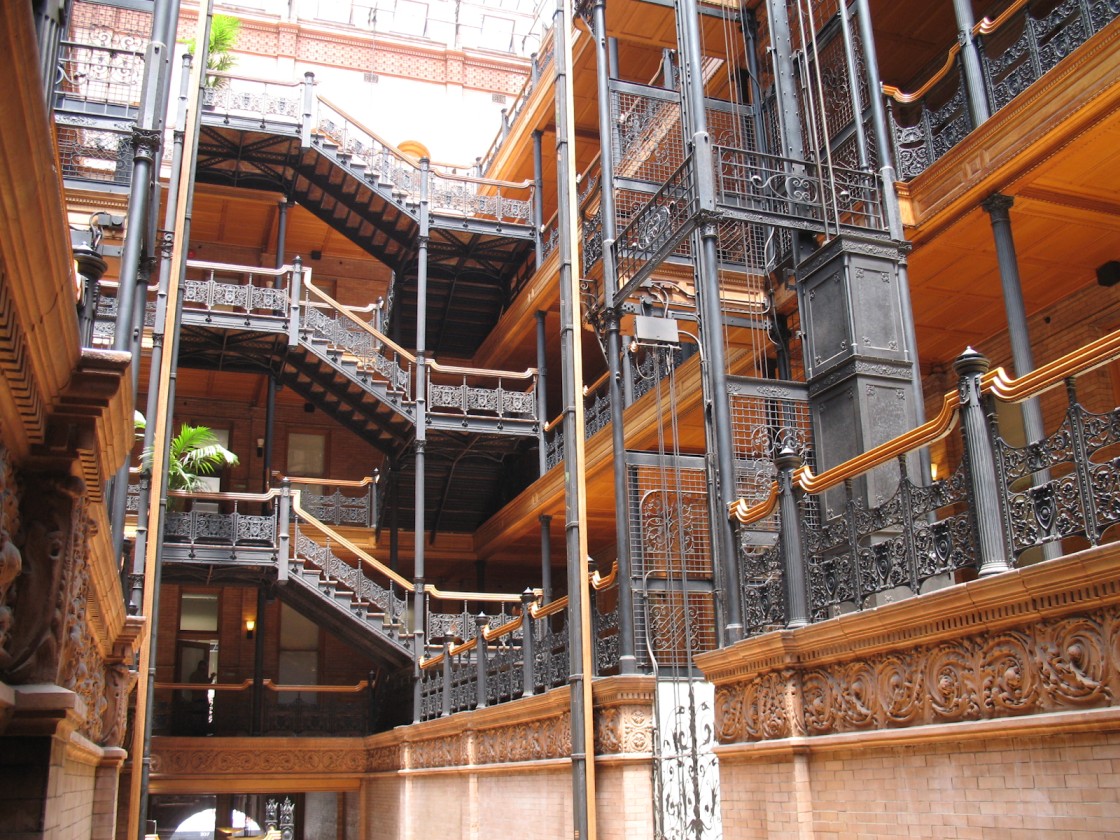This image captures the interior of a multi-level building, possibly an apartment or hotel, characterized by a distinctive arrangement of staircases and rich architectural details. The building features multiple staircases with brown wooden tops and silver side railings, embellished with gold accents on the banisters. Situated at the center is a black, metal-caged elevator, revealing its strings and a white base, adding to the vintage aesthetic. The walls are predominantly brown wood and stone, contributing to the warm, earthy ambiance, with black wrought iron elements underneath the staircases. The ceiling also displays the same brown wood, reinforcing the cohesive décor. The lower part of the image shows a doorway framed in brown with adjacent windows and lit fixtures, adding a welcoming glow. Verdant plants in flower pots accentuate some of the floors, alongside a person standing in the doorway at the bottom left of the image. The overall scene is a blend of design elements, from the concrete and brick walls at the bottom to the intricately detailed staircases and woodwork, capturing the essence of a thoughtfully crafted interior space.